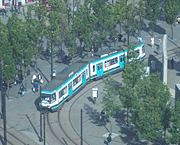The image is a small, inch-and-a-half square photograph displaying a train ride reminiscent of those at amusement parks, possibly Disneyland. The train is composed of several blue, aqua blue, and white cars with black roofs, captured on tracks meandering through a park-like setting. Despite the photo's fuzzy and slightly blurred quality, details reveal lush, green trees prominent in the upper and lower right sections. The track appears to traverse a concrete area, suggesting a public space where people might walk around and shop. The foreground includes small specks of people and tall poles, bordered by a fence. The scene unfolds under bright, sunny skies, indicating a clear day with no snow present.